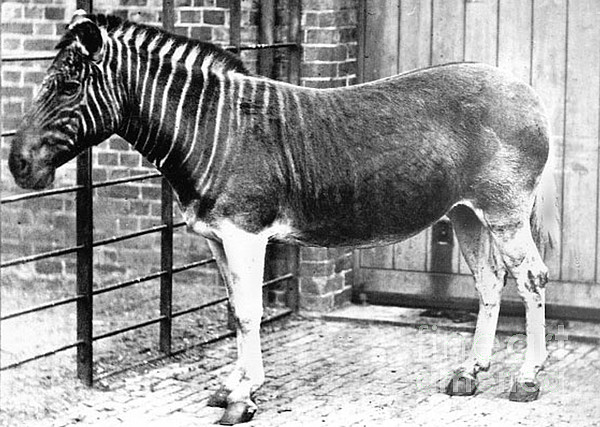The black and white photograph depicts a zonkey, an intriguing hybrid animal that has a zebra-like head and neck adorned with distinct black and white stripes, while its body transitions into a solid brown color, resembling that of a donkey. The zonkey's mane is stiff and bristly, standing erect on its head. Its legs appear white, possibly due to the lighting or camera settings, and it stands on a floor made of bricks. The zonkey, about the size of a pony, is positioned leftward in the image, enclosed within a tall black metal fence situated in an open stall setting. The background consists of a rustic scene with a brick wall on one side and a wooden wall on the other, complemented by a wooden floor, creating a barn-like atmosphere.